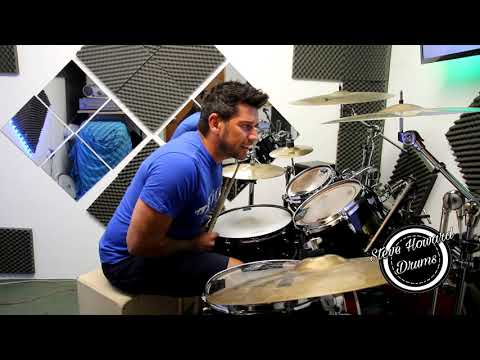The image features a white man with dark, spiky hair and light facial hair, seated on an off-white stool while leaning over a black drum set with drumsticks in his hands. He wears a medium blue short-sleeve t-shirt with white writing on it and dark shorts. The man appears to be engaged with something off-screen to his right, perhaps reading music or conversing, as his mouth is slightly open. The room’s walls are adorned with acoustic panels in a mix of black checkerboard and eggshell patterns, interspersed with large square mirrors composed of smaller square sections arranged in a diamond pattern. The photograph itself is bordered by black at the top and bottom, and features a logo in the lower right corner: a black circle encompassing a white circle with black text reading "Steve Howard Drums" in diagonal white print.